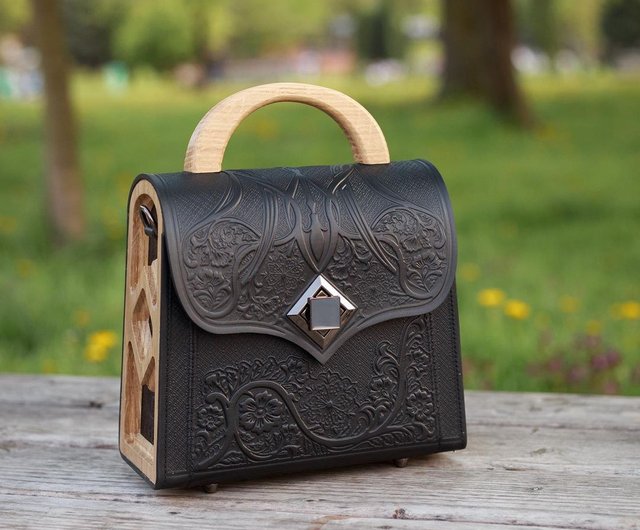A perfectly square photograph depicts a stylish purse stationed upright on a light wood table or bench, set against a blurry, park-like background featuring green hues, tree trunks, and touches of yellow flowers. The purse, predominantly black with an intricate floral filigree design, is the focal point. It features a wooden semicircular handle at the top, the same light shade as part of the purse's side panel. The purse's side panel arches gracefully, echoing the handle's curve, and there's a distinctive diamond-shaped cutout. The front flap, matching the arch, folds halfway down and fastens with a square, silver metal clasp that operates by turning 45 degrees to secure.